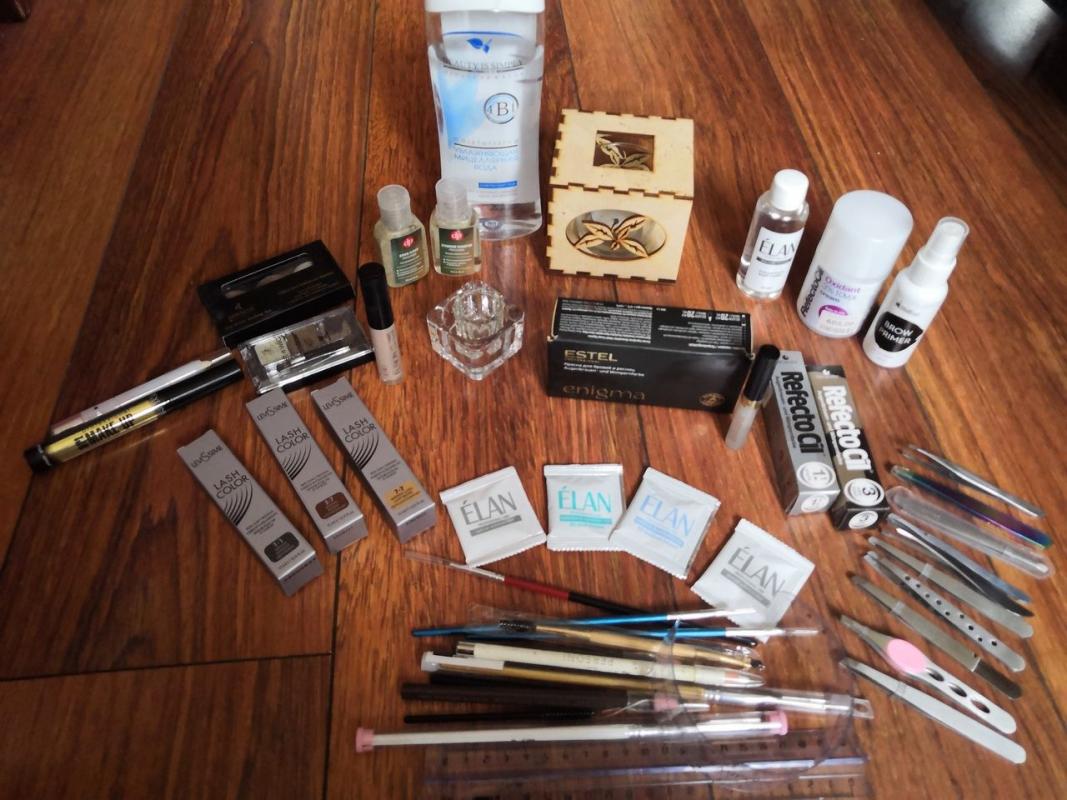On a rustic wooden table, a variety of makeup implements, liquids, and materials are meticulously arranged. In the back row, two containers hold an unknown liquid, possibly disinfection gel or nail polish. Next to them, on the right, stands a transparent bottle filled with an indeterminate fluid. Adjacent to this is a carved wooden box featuring an intricate floral design. Further to the right, three distinct bottles display their unique beauty products, with one clearly identifiable as a small white spray bottle labeled "Brow Primer" in white text on a black circular background. In front of these items, three silver boxes labeled with lash colors in black, brown, and beige hues are neatly positioned. Four packets of wipes, from the brand Elan, are also visible. Scattered among these items are numerous tweezers and other makeup tools, completing the detailed scene of a well-equipped makeup station.